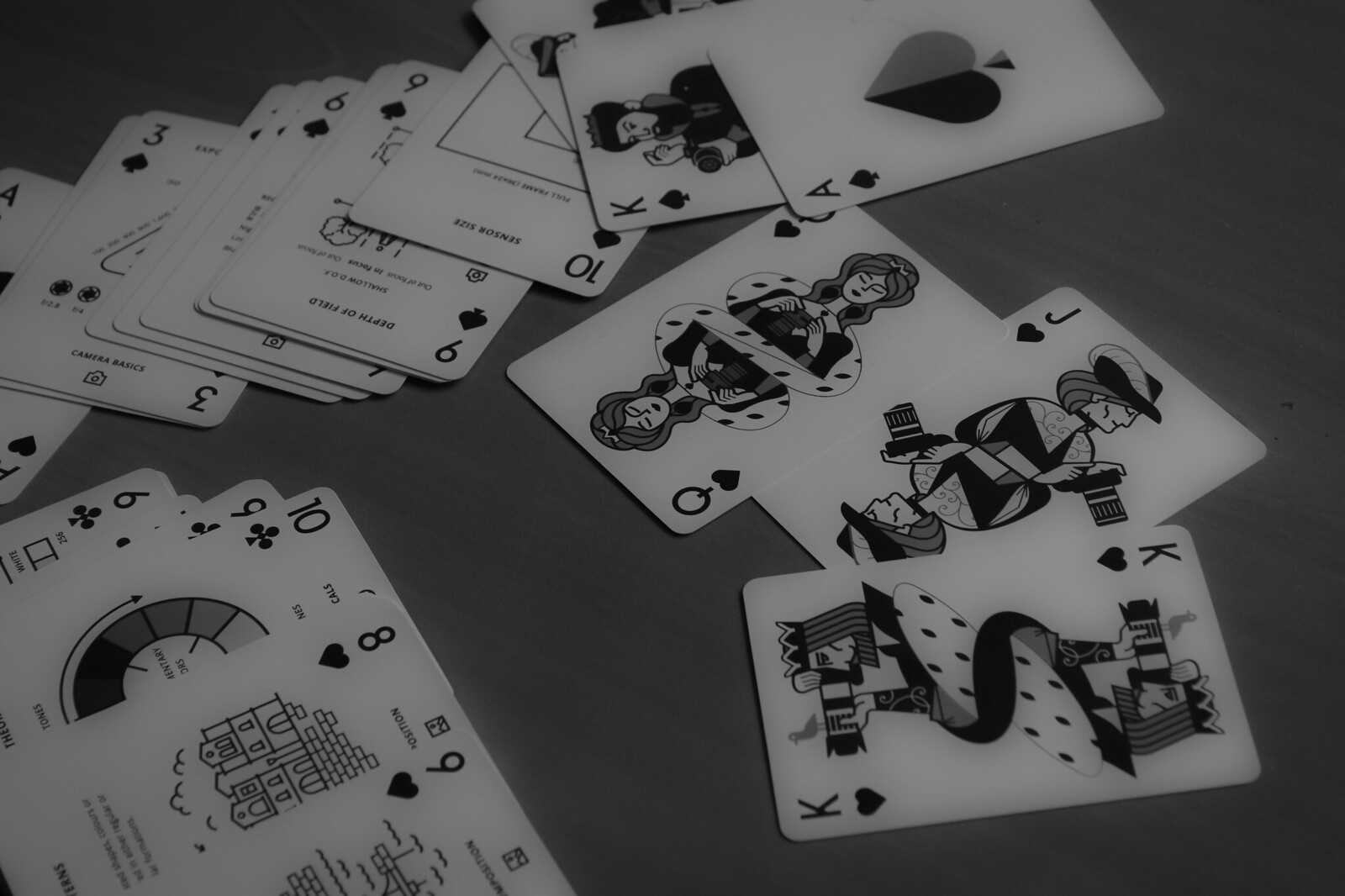This black and white photograph captures an array of playing cards neatly arranged in various upright stacks. Closest to the camera, prominently displayed, are the Queen, Jack, and King of Hearts, each showcasing intricate mirrored imagery. The Queen, with her dark hair adorned by a crown, wears a white shawl with black spots and holds a cup, presumably golden, in her hand. This Queen's image is mirrored identically below on her card. The mirrored design is characteristic of the face cards in the foreground. Above these three Hearts cards lies another pile, crowned by the Ace of Spades, which deviates from the mirrored design as it features a singular depiction. In the background, other cards are visible, scattered in different orientations and displaying a range of numbers such as sixes, nines, threes, and fours, each with its own unique imagery.